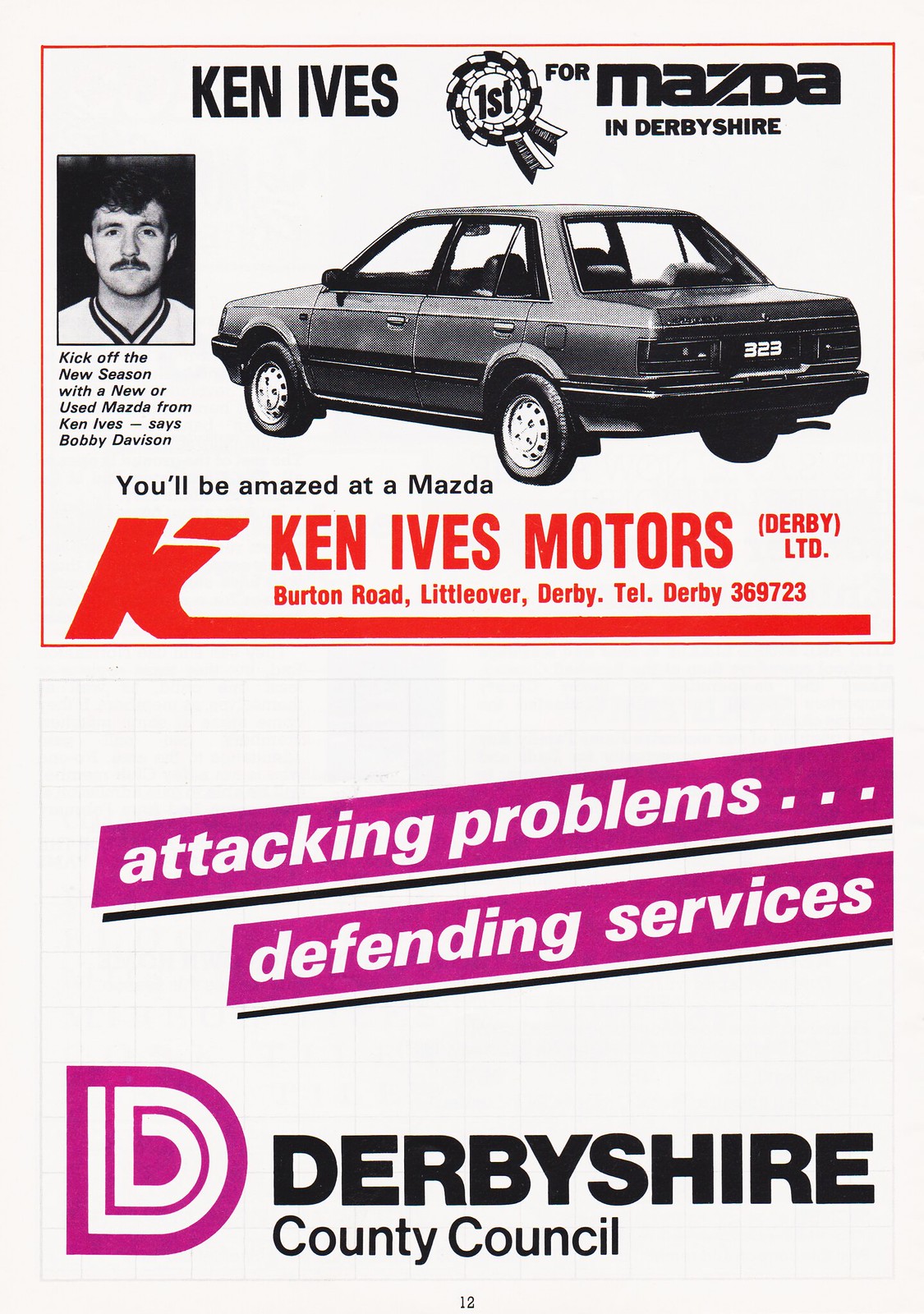The image is an advertisement from what appears to be a newspaper or magazine from the 1980s or early 1990s, featuring Ken Ives Motors, a Mazda dealership in Derbyshire. At the top, the advertisement prominently displays the name "Ken Ives" along with an award pin that reads "First for Mazda in Derbyshire." Below this, there is a black-and-white photograph of an older style Mazda and a portrait of a man with a mustache and curly hair, identified as Bobby Davison, who endorses the dealership with the slogan, "Kick off the new season with a new or used Mazda from Ken Ives." The ad also includes the catchphrase "You'll be amazed at a Mazda." Further down, detailed contact information is provided in red font: "Ken Ives Motors, Derby LTD, Burton Road, Little Over, Derby. Telephone: Derby 369723." At the bottom of the page, a purple banner carries a message from the Derbyshire County Council, stating "Attacking problems...defending services," alongside a large purple "D" and the words "DERBYSHIRE CITY COUNCIL" in black capital letters.